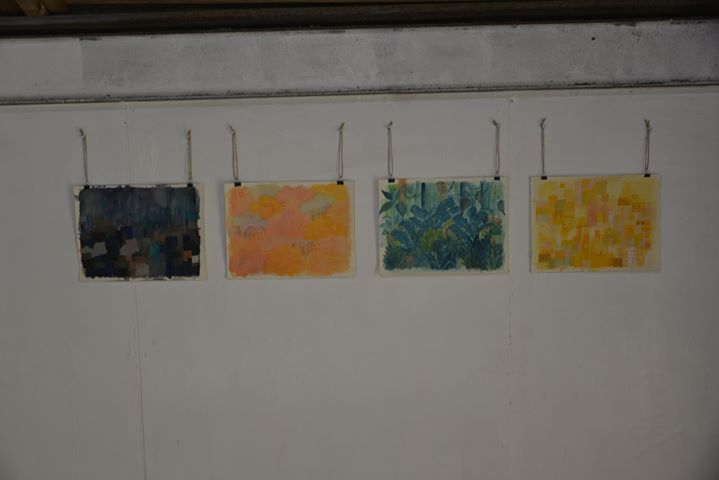This image displays a series of four paintings suspended on a plain white cinder block wall, featuring a black strip running along the top near the ceiling. Each painting is hung by two pieces of string attached to nails or thumbtacks, with strings originating from the top left and right corners of the paintings. The artworks are all the same size, reminiscent of standard A11 sheets, and exhibit abstract themes and colorful palettes.

From left to right, the first painting presents shades of purple and black, forming an abstract composition. The second painting, predominantly in hues of yellow and orange, features abstract forms and contains small white ovals resembling clouds. The third painting uses a blue and green color scheme with discernible plant elements, such as leaves. The fourth and final painting to the right combines greens, oranges, and yellows in an abstract manner, accentuating overlapping square forms.

Overall, the paintings share a minimalist yet vibrant aesthetic, unified by their method of suspension and the stark white backdrop that highlights their colors and abstract forms.